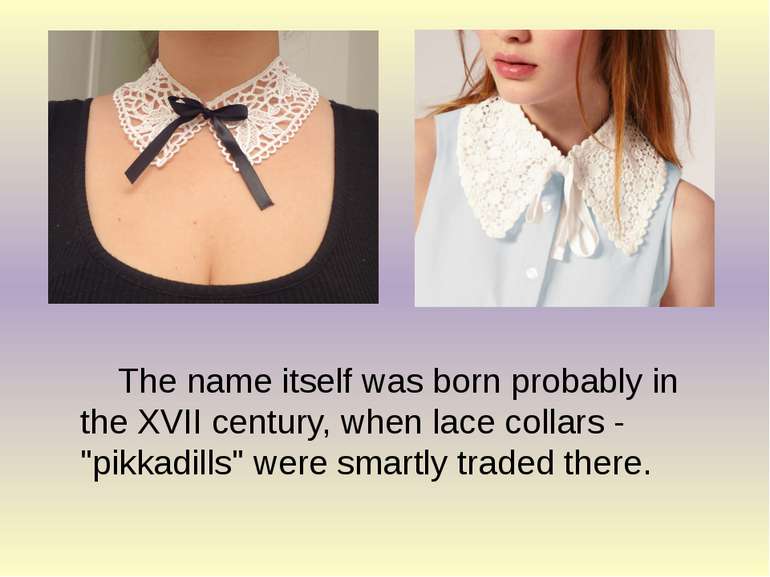The image features a PowerPoint slide with a pastel gradient background, transitioning from pale yellow to purple and back to yellow. Centered at the bottom is black text that reads, "The name itself was born probably in the XVII century when lace collars, picadilles were smartly traded there." The upper part of the slide contains two squares displaying photos of young women modeling lace collars, also known as picadilles. The women are shown from the chest up, with the woman on the left wearing a low-cut black top with a white lace collar and a black ribbon tied into a bow. The woman on the right, captured up to her nose, sports a light blue buttoned vest and a larger white lace collar with a white ribbon bow. The slideshow slide showcases the historical evolution of these lace collars from the 17th century to the present.